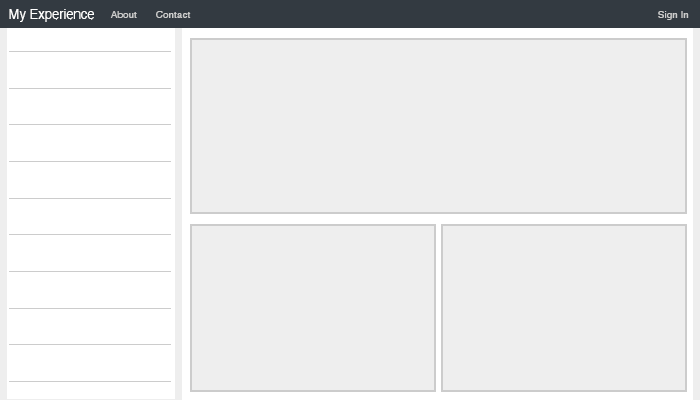The image appears to be a screenshot of a website builder interface. At the very top right, the word "Sign-In" is displayed in white text. To the far left of the top, "My Experience" is prominently featured in bold white text, with "About" and "Contact" appearing to its right in a smaller, unbolded font. The background at the top of the image is a dark blueish black, adding contrast to the white text. 

Beneath the top left section, several thin horizontal lines extend vertically downwards, flanked by vertical rectangular boxes in a light gray color. These lines and boxes are set against a white background, suggesting a layout or grid system.

In the middle right section of the image, three boxes are arranged. The topmost box is larger and shares the same light grayish color as the two smaller boxes positioned directly beneath it. Additionally, another vertical rectangular light gray box is situated along the far right edge of the image. The overall design features a minimalist aesthetic with a clear emphasis on a structured layout.